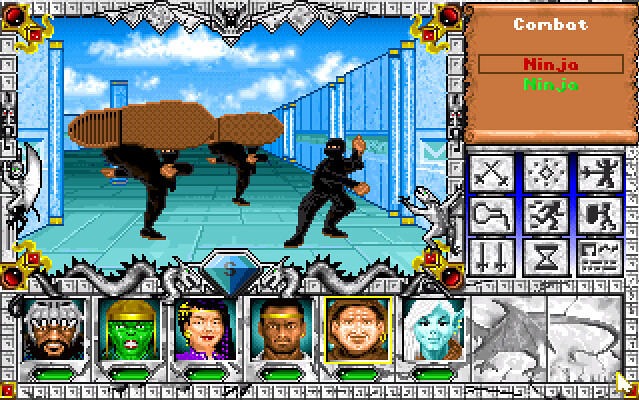In this vibrant screenshot from a computer game, the image's right quadrant prominently features a brown banner box labeled with the words "combat" and "ninja" twice. Along the bottom edge of the game interface, small white squares form a continuous border that extends upwards. Positioned above this row of squares are character portraits, seemingly representing potential opponents or playable characters. The first portrait is of a Black man partially obscured by a face covering. Adjacent to him is a character adorned in what appears to be a green-colored pharaonic headdress. Next is a woman with distinct black hair, followed by another Black man. Subsequent to these characters is a white man sporting a brown hat and hoodie. The final character stands out as a blue elk with prominent pointy ears and striking white hair. Dominating the main part of the screen are detailed scenes of ninja combat, with noticeable shoe prints covering the heads of two characters, hinting at dynamic movement and action in the game.